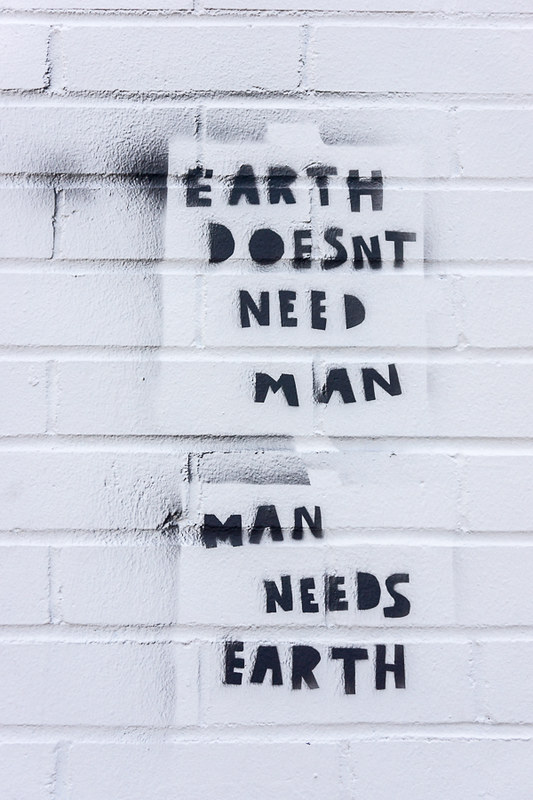The photograph showcases a white-painted brick wall adorned with a black, spray-painted message formed using stencils. Two slightly brighter white rectangles, arranged one above the other, contain the bold, hand-cut text. The top rectangle reads, "Earth doesn't need man," while the bottom one states, "Man needs earth." Evidence of overspray highlights the stencil's outline, especially noticeable around the word "Earth." The distinct contrast in shades underscores the method used to deliver the poignant environmental message.